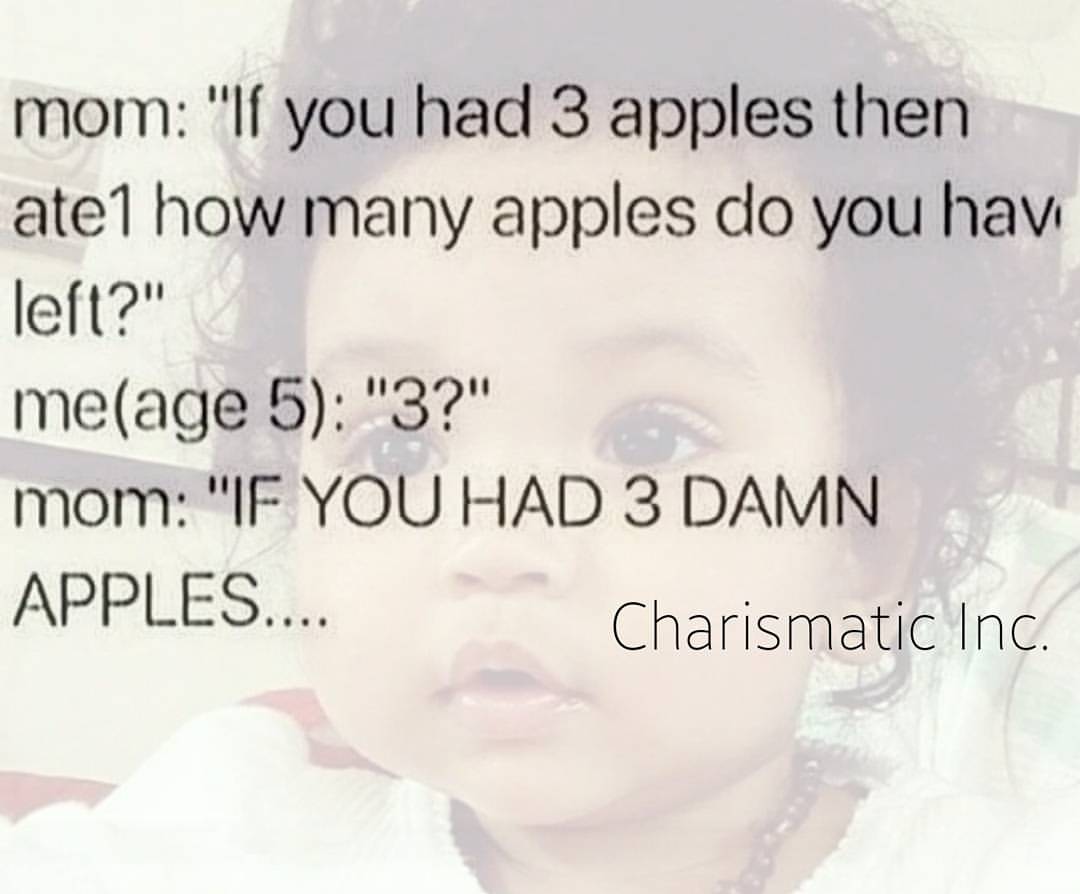In a meme-style image circulating on social media, there's a light, semi-opaque background featuring the face of a young child with curly, messy hair, brown eyes, and black eyebrows. The child, captured wearing a white shirt and a bead necklace, gazes directly at the camera with a thoughtful expression. Overlaying the image is a humorous conversation between a mother and her 5-year-old child. The text, written in black, reads: 

"Mom: If you had three apples and ate one, how many apples do you have left?
Me (age 5): Three.
Mom: If you had three damn apples..."

In the bottom right corner, the text “Charismatic Incorporated” can be seen. 

The meme humorously captures the child’s persistent misunderstanding of basic arithmetic, encapsulating a typical yet endearing moment between a parent and a young child.